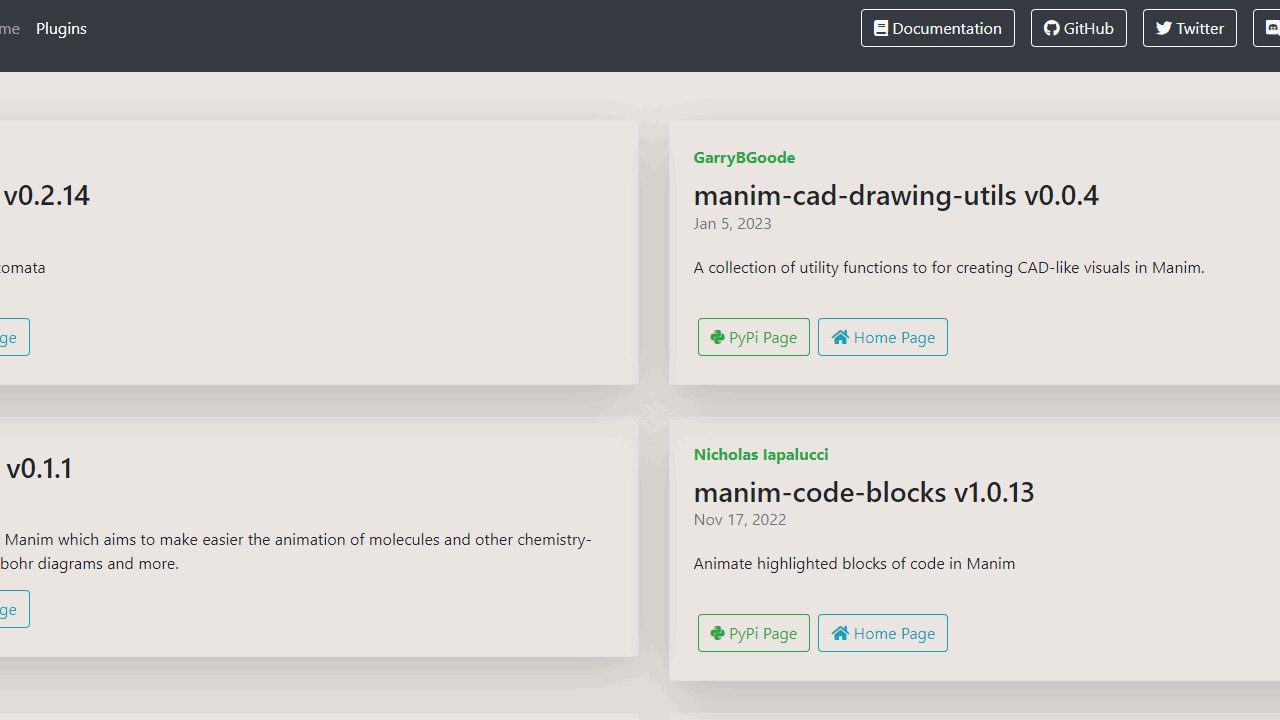A fast-scrolling GIF screenshot captures a dynamic view of a user interface showcasing various plugins. The interface predominantly features a dark gray background with mid-gray, 3D-raised, rectangular sections on both the left and right sides. At the top, there's a navigation bar including clickable buttons labeled "Documents," "GitHub," "Twitter," and another partially visible option. 

The scrolling begins, revealing categories such as "Plugins," "Editor," "CAD," "Drawing," "Code," and "Editor Chrism." Each plugin entry includes a name and is accompanied by functional buttons. Some entries feature a green "PyPI page" button with a green plus icon, possibly indicating an option to visit a Python Package Index page or add the plugin. Other entries display a blue "Home Page" button, bordered or backed in blue. Version numbers are listed alongside each plugin, such as "Version 0.04," "Version 6.42," and "Version 1.013."

Due to the rapid scrolling speed, extracting more specific details is challenging, but the overall layout hints at a comprehensive plugin management system with easy navigation and clear categorization.